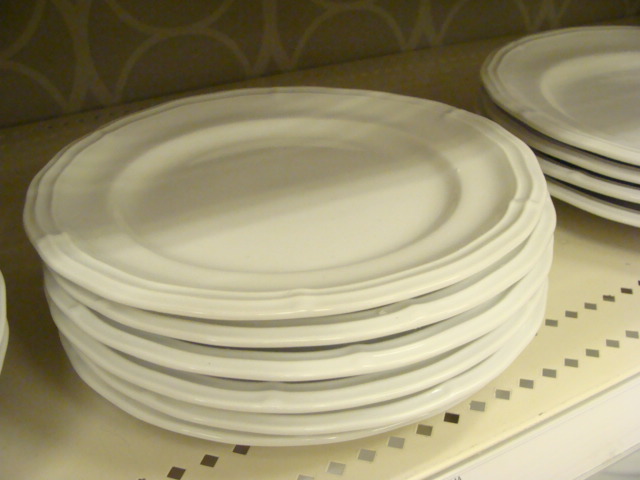The image is a color photograph showcasing a close-up view of a metal shelf in a retail store. The shelf features a distinctive design with two rows of small diamond-shaped cutouts along its front edge. The back wall behind the shelf appears to be light green or possibly gray, adorned with a white circular or dotted pattern.

The primary focus of the image is a stack of white dinner plates prominently positioned on the shelf. The main stack consists of six circular plates, each with a recessed center and a slightly scalloped, ridged border. To the right of this main stack, near the upper right part of the photo, there is another stack of four similar plates. Additionally, a hint of another stack can be seen on the left side, vaguely visible with the edge just peeking into the frame, casting a subtle shadow on the main stack.

The plates, while plain, possess subtle decorative elements in their ridges, adding a touch of elegance to their simple design. The metal shelf with its punched diamond design and the patterned wall together create a visually interesting background for the otherwise unremarkable white plates.